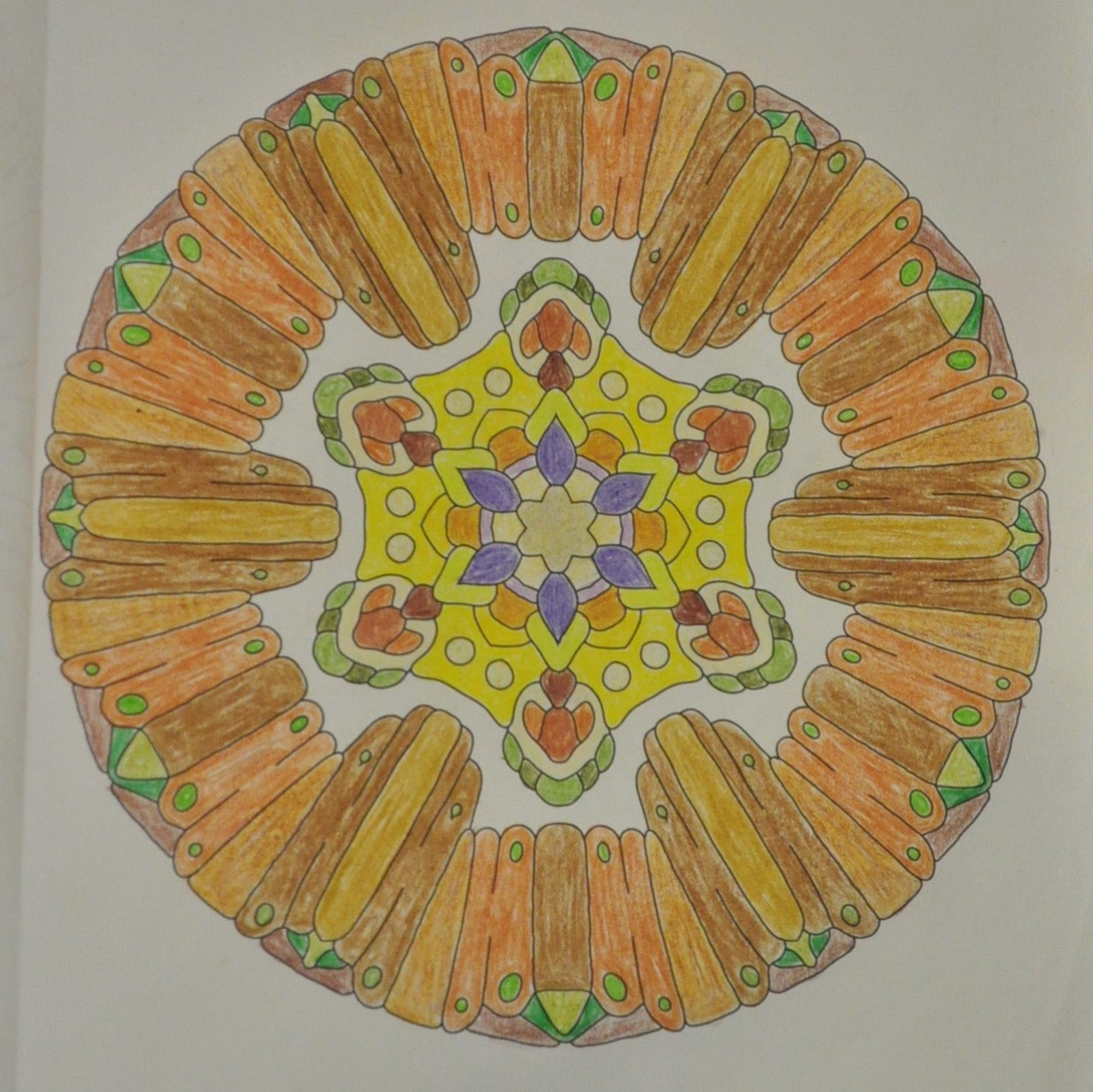This hand-drawn image features a wreath-like structure encircling a kaleidoscope center. The wreath is crafted from objects resembling pencils and popsicle sticks or tongue depressors, meticulously arranged in a circular pattern. Within this arrangement, six larger elements stand out at approximately the 11, 1, 3, 5, 7, 8, and 9 o'clock positions. The wreath part showcases a palette of brown and tan hues, adorned with green dots and circles, adding a touch of vibrancy.

At the heart of this whimsical wreath lies a kaleidoscope image characterized by its intricate six-point symmetry. The kaleidoscope features green points interspersed with tiny jet-like shapes within white circles, and brown ovals, creating a visually engaging pattern. The center radiates with shades of yellow and orange, serving as a warm focal point. Complementing this is a cluster of six purple, fleur-de-lis-shaped leaves that project outward from a central six-point star. This convergence of colors and shapes results in a mesmerizing and intricate design.